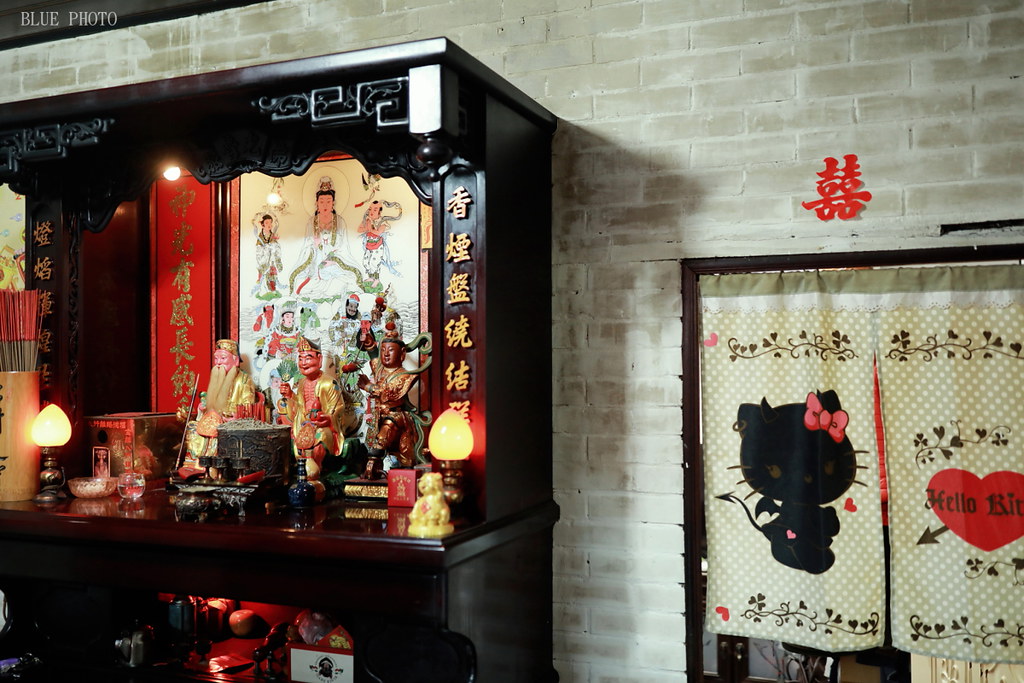The image depicts the interior of a room with a distinct Asian cultural theme. The back wall features a pattern resembling gray and white bricks. On the left side of the image, there is a dark brown wooden altar decorated with numerous statues and figurines, including various representations of Buddha and mythological figures. The altar is intricately detailed with engravings of Chinese or Japanese characters running vertically along its edges, and two lamps illuminate the scene. To the far left of the altar, a canister holds a collection of red and gray incense sticks.

On the right side of the image, a doorway is partially obscured by a curtain. The curtain is adorned with a depiction of Hello Kitty, the iconic black cat with a pink bow, along with a heart shape that also bears the Hello Kitty logo. Above the doorway, another red Japanese or Chinese symbol is visible, adding to the room's cultural ambiance.